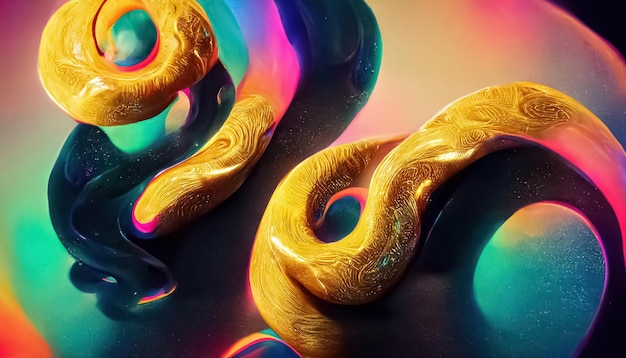The image depicts an abstract artwork with a mesmerizing array of vibrant colors and shapes. The composition features what looks like sinuous, snake-like forms that twist, bend, and intertwine in a liquid-like, almost half-solid, half-liquid appearance. The artwork incorporates elements that mimic polymer clay, resin, amber, and glass, with a striking presence of fluorescent pink and neon colors. Black glass shapes fold and warp into intricate, circular patterns, adding depth and shadow to the piece. One prominent snake-like form coils in the upper left corner, while another stretches diagonally across the center towards the right. The varied hues—including yellow, green, red, and black—create a lively and random visual experience, making the piece appear almost as a computer-generated illustration devoid of people, writing, or recognizable structures. The image captures the essence of abstract art with its dynamic interplay of colors and irregular, organic shapes.